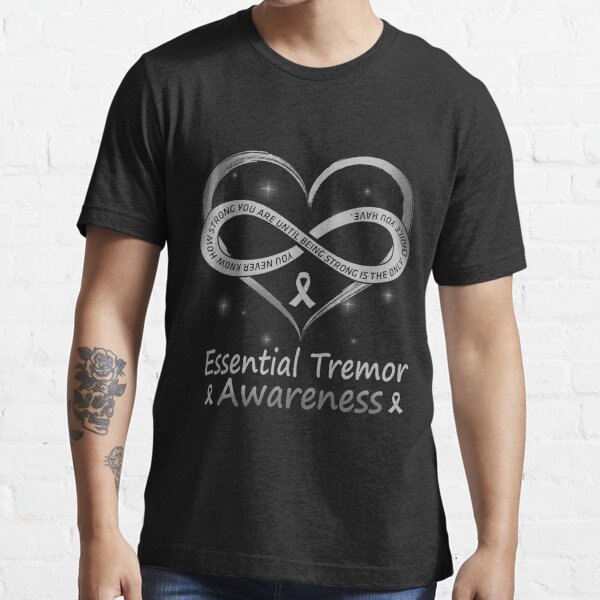The photograph showcases a man modeling a black t-shirt, standing in front of a white brick wall. The t-shirt prominently features a design at its center, including a white heart containing an infinity symbol. Inscribed within the infinity symbol is the phrase, "You never know how strong you are until being strong is the only choice you have." Beneath the heart and infinity symbol is the phrase "Essential Tremor Awareness," flanked by ribbons on both sides. The man, visible from neck to hips, has tanned skin and a tattoo on his right forearm, which appears on the left side of the image. The tattoo depicts a skull adorned with flowers. The photograph has the appearance of an online product listing, likely intended to promote awareness for essential tremor.